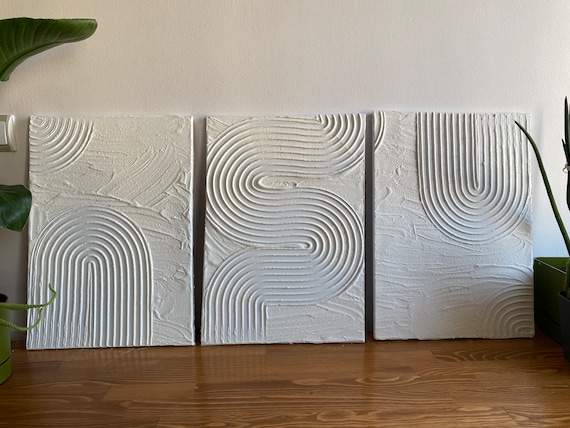This photograph showcases a set of three minimalist 3D canvases, all leaning against a pristine white wall. Each white canvas presents an intricate texture, reminiscent of zen garden patterns etched with a stick. They are carefully displayed on a shiny wooden surface. Starting from the left, the first canvas features a looping design concentrated on the bottom left corner, forming an upside-down U-shape that extends outward. The middle canvas showcases an elaborate S-shaped pattern that traverses the entire surface from top to bottom. The third canvas on the right displays a loop that begins from a thin U-shape in the middle, expanding into wider arcs, reaching the top right corner. The artwork, appearing almost sculptural, captures the essence of fluid, swirling lines, providing a serene and cohesive visual experience.